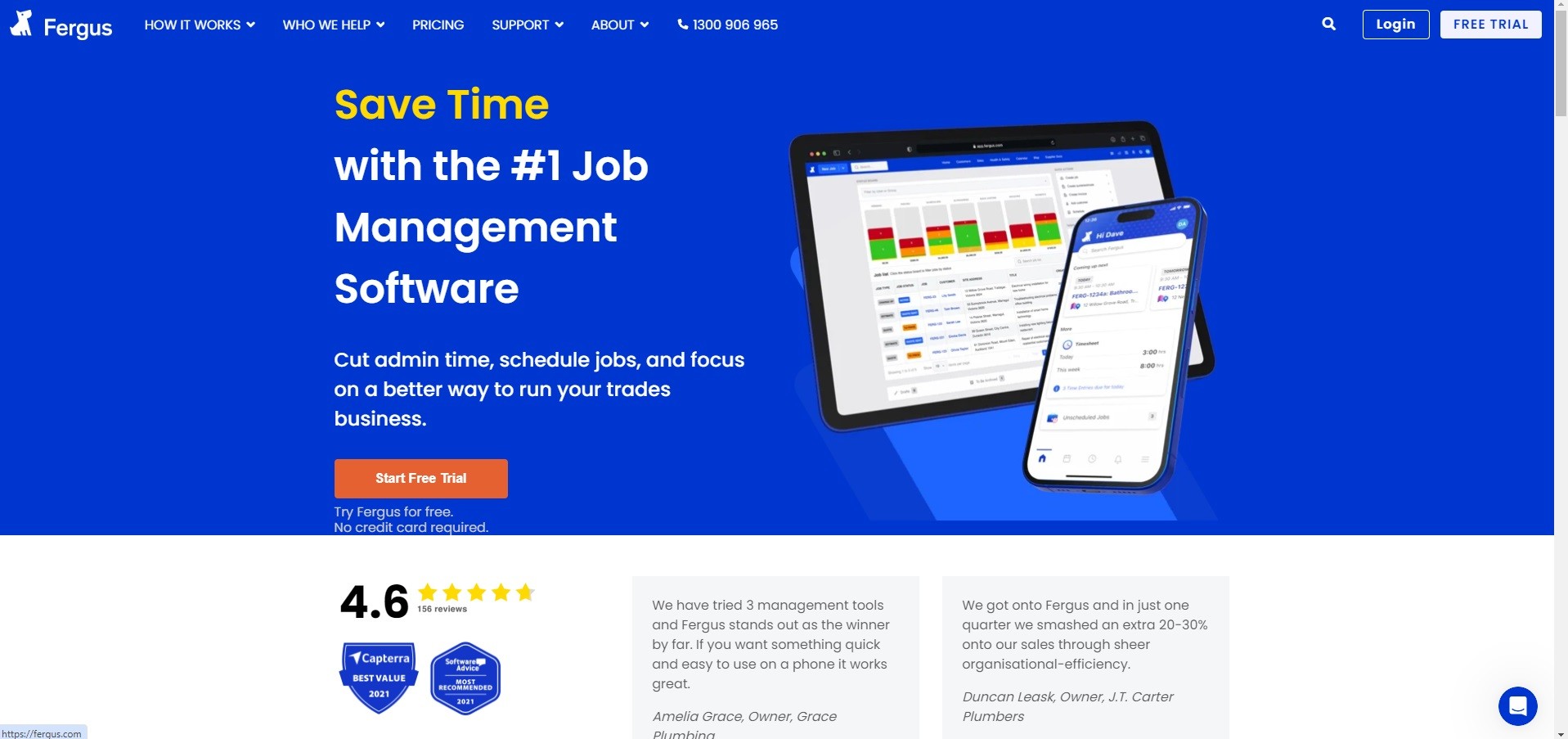The screenshot captures a page from the Fergus website with a royal blue background. On the top left in modestly-sized white letters is the word "Fergus," accompanied by a tiny cartoon figure of a small dog. To the right of the "Fergus" logo are several dropdown menus labeled “How it works,” “Who we've helped,” “Pricing,” “Support,” “About,” and a call number for customer inquiries. Farther to the right, a search bar is prominently displayed, followed by “Login” and “Free Trial” buttons.

The central image shows a tablet and a phone displaying the Fergus application. Above these devices, bold yellow text reads "Save Time," followed by a declaration in white that Fergus is the number one job management software. Beneath this, additional text emphasizes that Fergus helps to cut administrative time, schedule jobs, and manage businesses more effectively. 

A standout orange button invites users to "Start Free Trial," with the assurance "Try Fergus for free, no credit card required." Below this call to action, the site shows informative sections that are somewhat vague by design, and highlights user satisfaction with a 4.6 rating from 156 reviews as well as two awards from 2021.